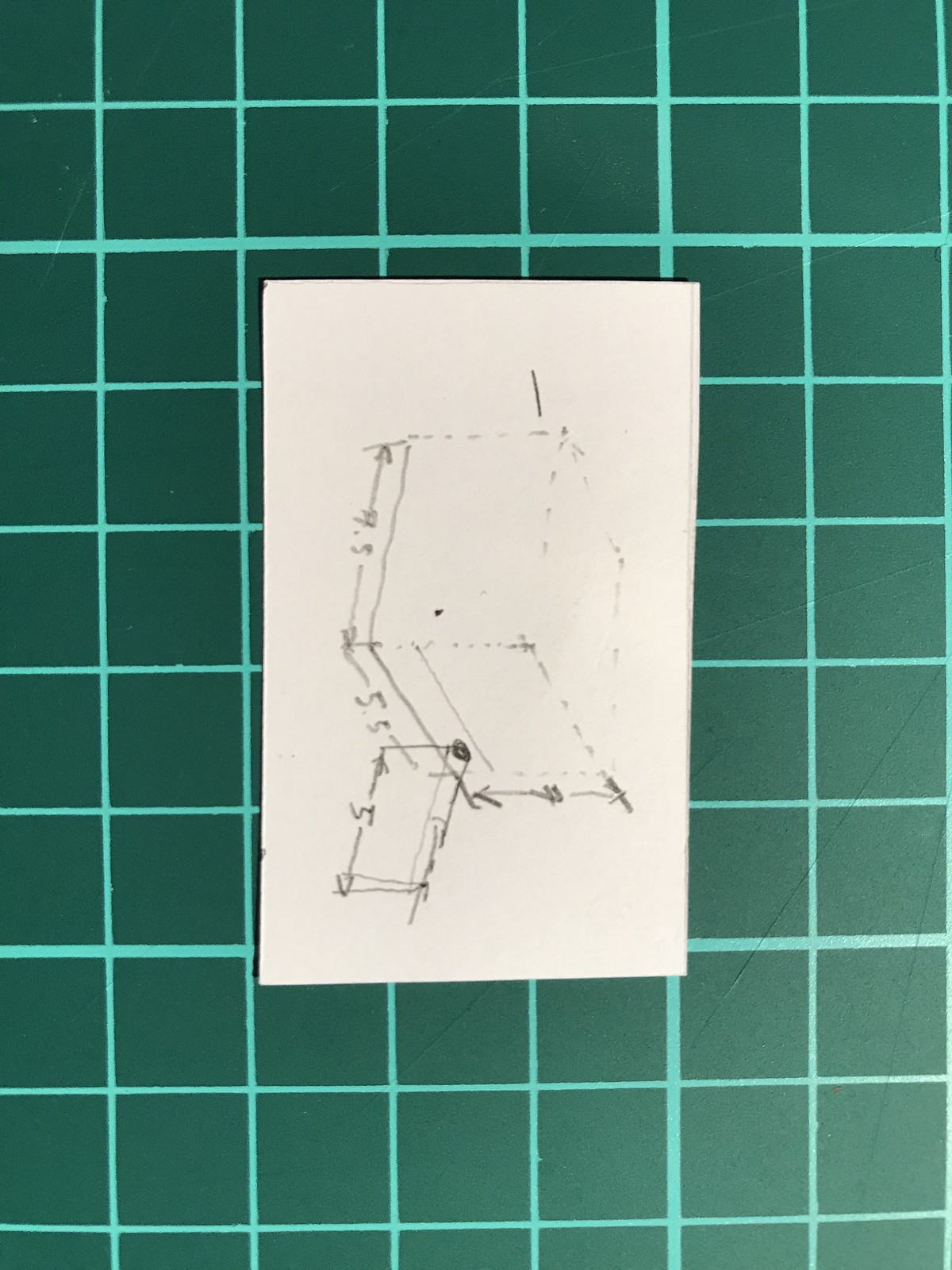A simple pencil sketch on white paper, dimensions approximately 3 inches by 5 inches, is placed against a dark green background. The background resembles a gigantic graph paper with horizontal and vertical yellow-green lines forming a grid pattern. The sketch, oriented sideways, appears to depict a basic architectural or construction plan, featuring a few walls and some handwritten dimensions, one of which is partially legible as "5x5". Located in the center of the paper, the drawing is accompanied by faint preliminary markings, suggesting the initial stages of design.